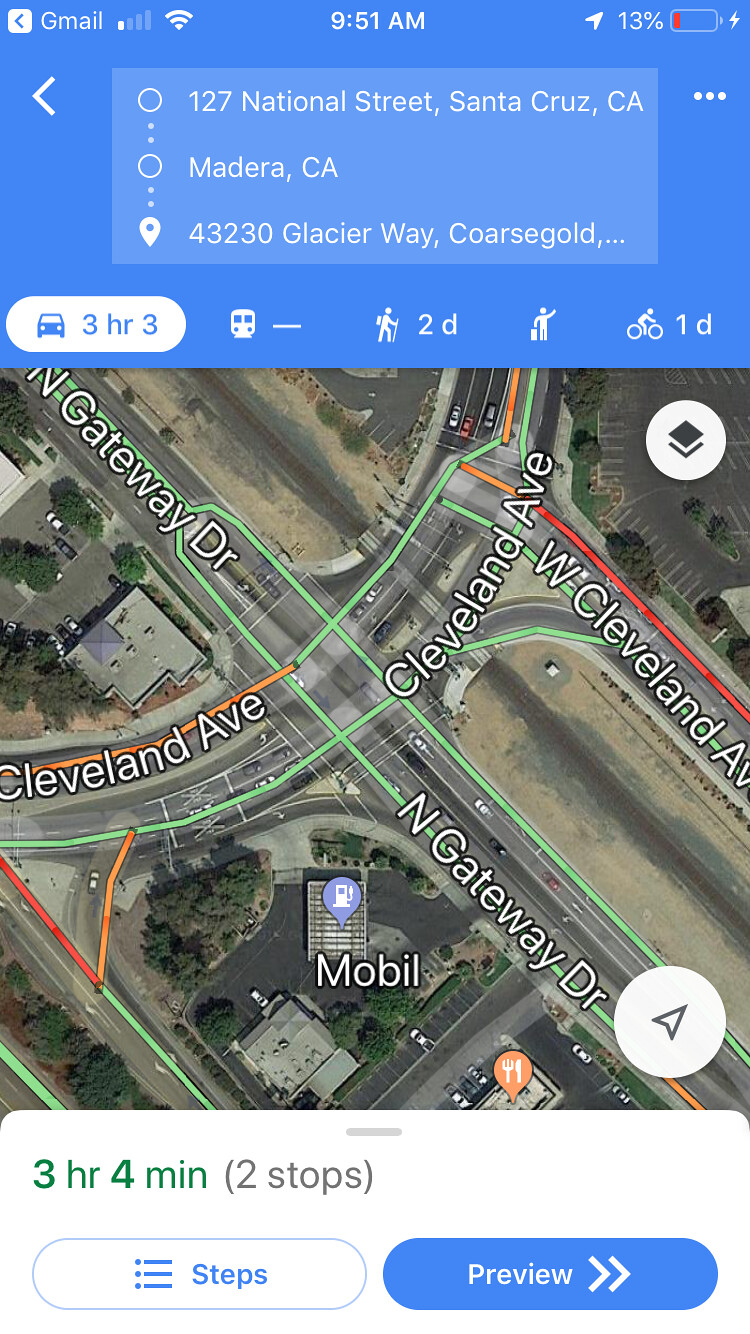A detailed caption for the described image could be:

"This is a detailed screenshot of a map application displayed on a cell phone. At the very top of the screen, a blue rectangle presents various status indicators: a Gmail icon, a low-level connectivity icon, and the current time, 9:51 AM, positioned centrally. Adjacent to these, an arrow icon points to '13%', highlighting the red battery indicator, signaling a very low battery level.

The map application is actively navigating a route from '127 National Street, Santa Cruz, California' to '43230 Glacier Way, Coarsegold, California', passing through Madera, California. The GPS estimates the travel time to be three hours and three minutes, and the mode of transport chosen is by car, as opposed to other available options like train, walking, rideshare, or bicycle.

The bottom half of the screen displays the map with street overlays in green, red, and orange colors, indicating various traffic conditions. Street names, such as North Gateway Drive and Cleveland Avenue, are clearly marked on the overhead satellite image. Additionally, a mobile gas station is identified on the map.

At the bottom of the screen, textual information indicates that the entire journey is expected to take three hours and four minutes, including two stops. Below this, two buttons offer further navigation options: a white rectangle with rounded corners labeled 'Steps', and a blue button to its right, labeled 'Preview' with two right-pointing arrows, both in white lettering."